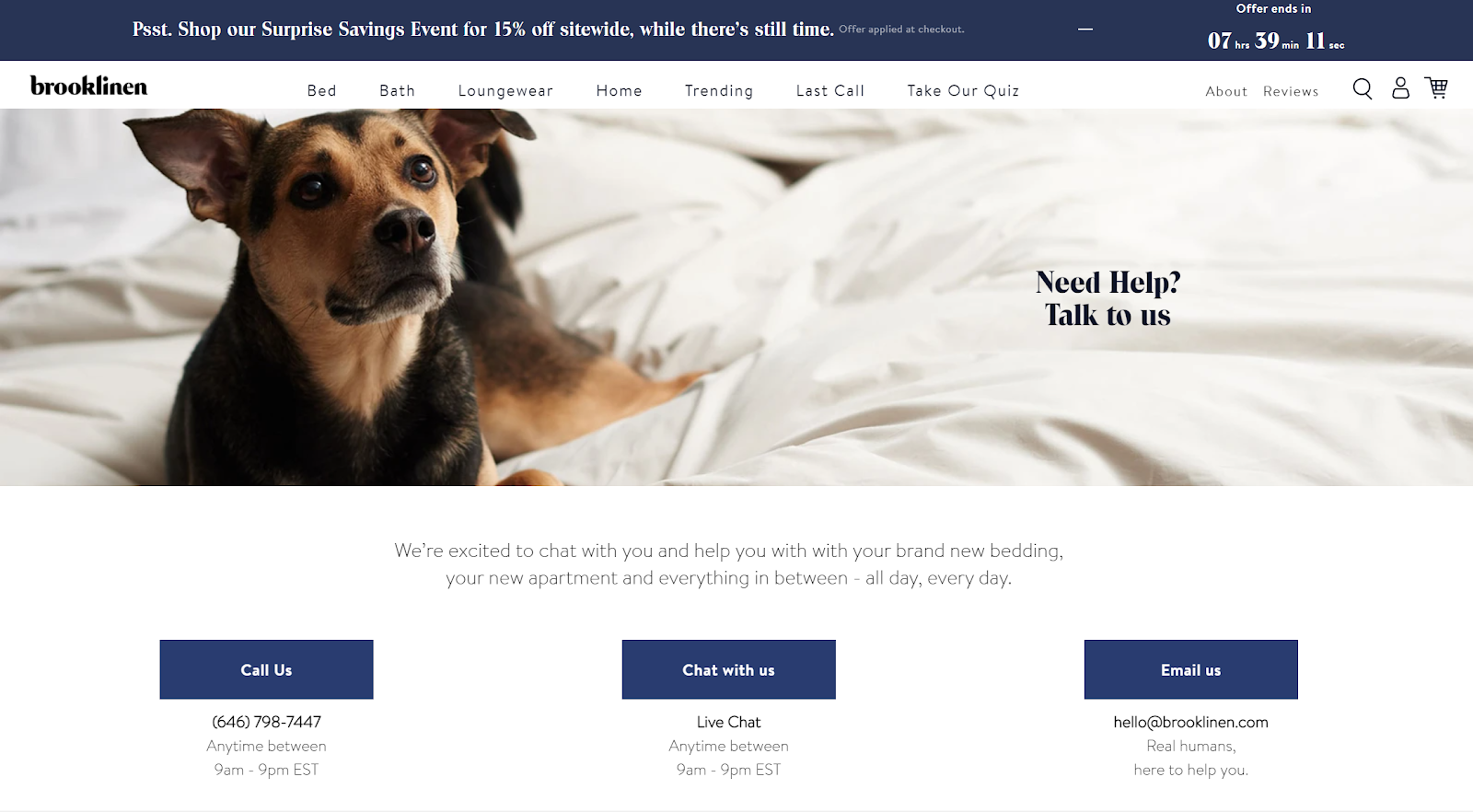**Detailed Caption:**

This is a screenshot of Brooklinen's main website page. Dominating the page is a large banner image depicting an adorable dog comfortably lounging on a neatly made bed and gazing directly at the camera. Superimposed over the bedcovers is the text, "Need help? Talk to us."

Above this main image, a prominent promotional banner highlights an ongoing offer: "Psst, shop our surprise savings event for 15% off site-wide while there is still time. Offer will be applied at checkout." The countdown reveals that the offer ends in 7 hours, 39 minutes, and 11 seconds.

The top navigation menu offers various categories for easy browsing. From left to right, the options are: Bed, Bath, Loungewear, Home, Trending, Last Call, and Take Our Quiz.

Beneath the main image, welcoming text invites customers to reach out for assistance with their new bedding, apartment setups, and more, available "all day, every day." 

Three interactive buttons provide different ways to contact the company:
1. **Call Us** - 646-798-7447, available between 9 a.m. and 9 p.m. Eastern Standard Time.
2. **Chat with Us** - Live chat available between 9 a.m. and 9 p.m. Eastern Standard Time.
3. **Email Us** - Reach out via hello@brooklinen.com, with real humans ready to assist.